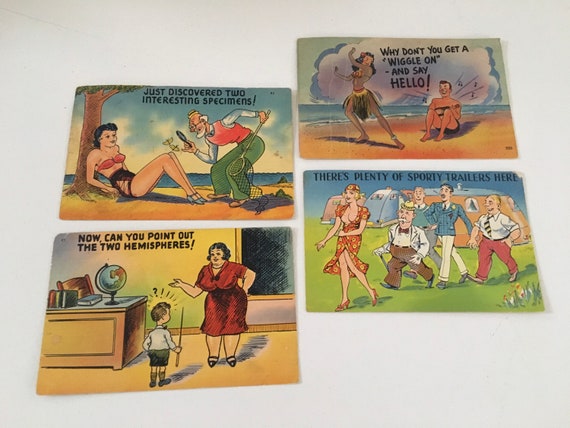This photograph features a flat lay of four vintage comic book-style illustrations set against a white background, appearing like products for sale. The images are arranged with two on the left side and two slightly higher on the right. 

In the top left, an older gentleman with a butterfly net and magnifying glass examines butterflies, one of which has landed on the knee of a woman in a 1950s-style bikini leaning against a tree. The caption reads, "Just discovered two interesting specimens."

Below that, the bottom left image depicts a woman in a red dress, presumably a teacher, engaging with a young boy holding a pointer and standing in front of a globe on a desk. The boy has a question mark above his head, and the caption asks, "Now can you point out the two hemispheres?"

In the upper right, a beach scene unfolds with a man seated and playing music, while a hula dancer performs nearby. The text above them says, "Why don't you get a wiggle on and say hello?"

Finally, the bottom right illustration shows a woman in a revealing orange dress walking across the grass, followed by three men. The backdrop features mid-20th-century style travel trailers, and the caption reads, "There’s plenty of sporty trailers here."